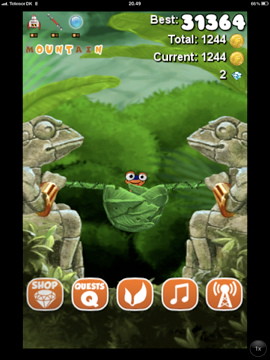This is a vibrant color photograph resembling a scene from a mobile game. At the bottom of the image are square icons with rounded edges, each featuring white symbols. These icons include a book, a music note, and a tower emitting radio waves. The main scene is dominated by a pair of frogs sitting on opposite sides, facing each other. Framed in the middle are a cluster of trees and what appears to be a body of water below. Unseen eyes peek out enigmatically from the trees, adding an element of mystery. Below the trees is a circular area resembling a basket woven from reeds. At the top of the image, white text displays the numbers "31364" on the right-hand side, with labels "total" and "current" next to coin symbols, indicative of the game's currency system. Additional smaller but unreadable icons are positioned at the upper left-hand corner.